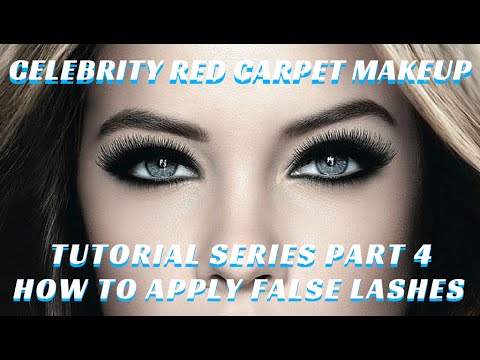This is a slightly low-resolution close-up image of a young woman’s face, primarily emphasizing her blue eyes. Her long, dark, likely false eyelashes and smoky eyeshadow draw immediate attention. She has brown, straight eyebrows with an arch at the ends and blonde hair framing her face on both sides, possibly dyed. The image is horizontal with black borders at the top and bottom. Over her forehead, in white letters with a blue drop shadow creating a 3D effect, it reads "Celebrity Red Carpet Makeup." Below her nose, divided into two lines, the text states "Tutorial Series Part 4" and "How to Apply False Lashes." The overall photo has a dim, monochromatic tone, adding a subtle focus on the makeup details being highlighted in the tutorial.